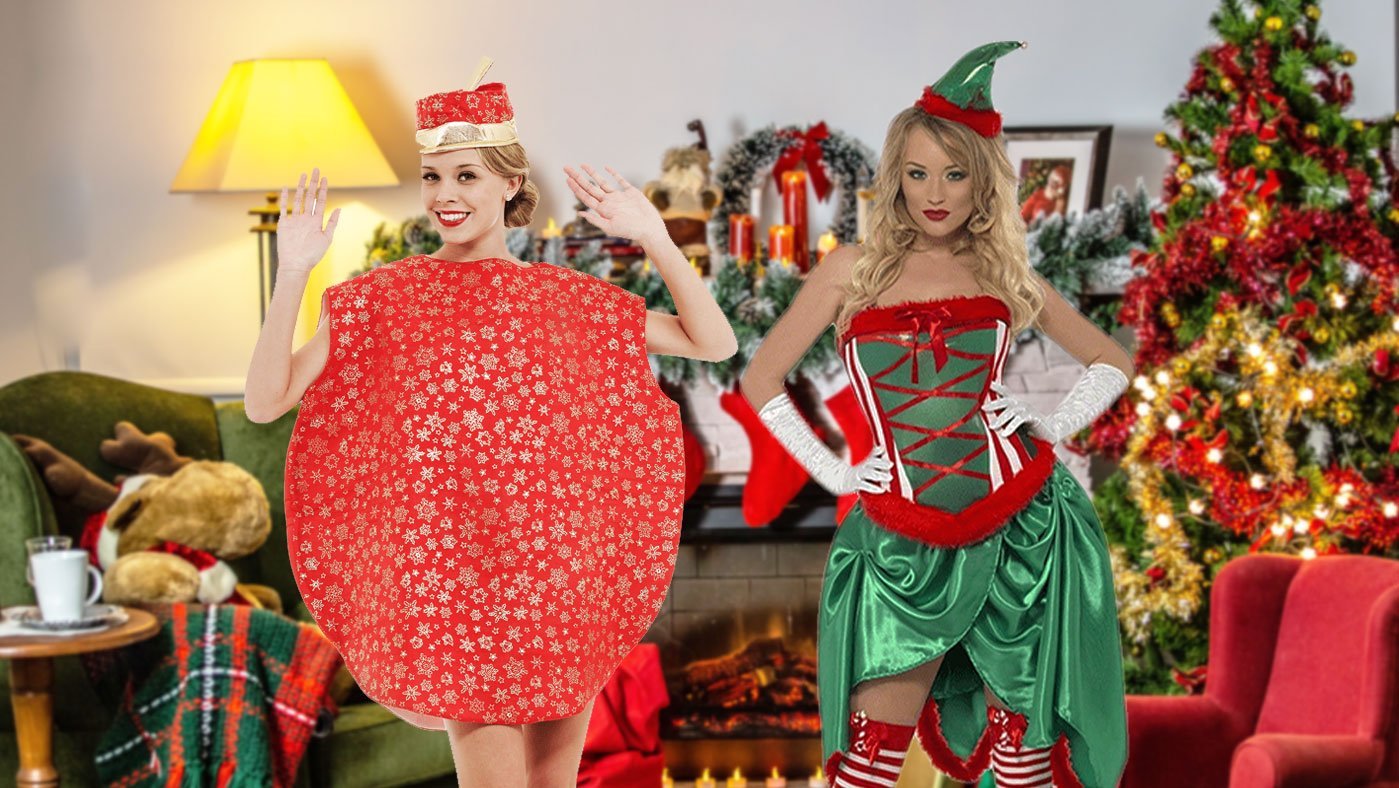In an indoor festive Christmas setting, two women are modeling holiday costumes in front of a decorated fireplace and Christmas tree. The woman on the left is dressed as a large, red Christmas ornament adorned with gold snowflakes. She stands with her arms up in a surprised gesture, and her costume includes a hat resembling an ornament cap with what looks like a wick, suggesting she might also represent a candle. The woman on the right is styled as a sultry version of Santa's helper, wearing a green corseted top with red ribbon and trim, a satin ruched skirt, red and white striped thigh-high stockings, white gloves, and a green elf hat with red trim. She has blonde hair and poses confidently with her hands on her hips, glancing sultrily at the camera. The background features a stuffed moose sitting on a cozy chair, stockings hanging above the mantel, and a Christmas tree decorated with red and yellow tinsel. Additional details include a glass of milk on an end table and a blurry assortment of photos on the fireplace mantel, enhancing the festive ambiance.